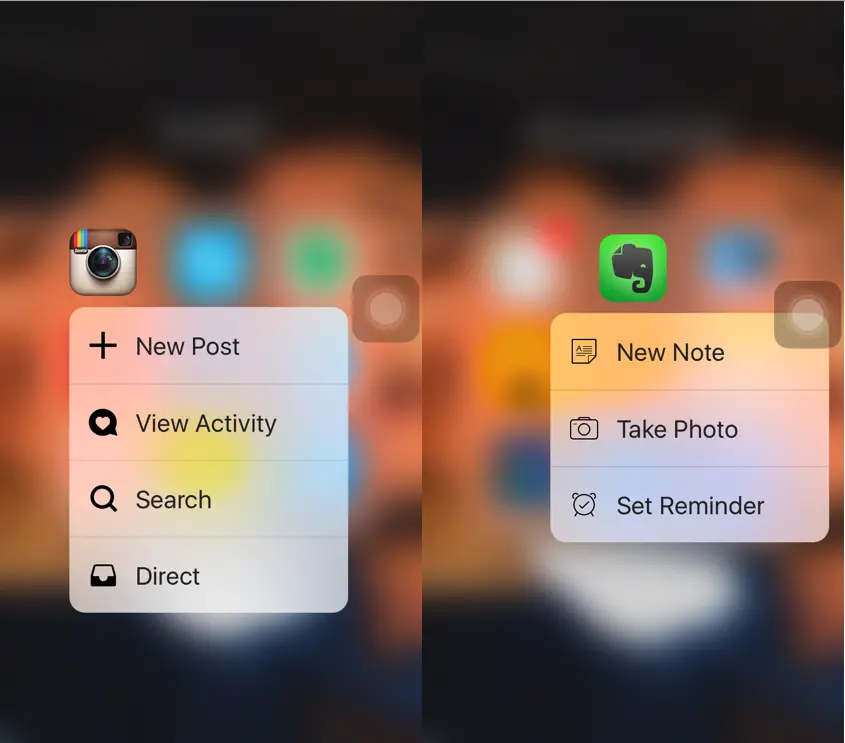The image consists of two side-by-side screenshots from a smartphone, each showcasing a different app interface. 

On the left screen, the background is notably blurred with black shading at the top and bottom, and a prominent orangish hue in the middle. Within this orange area, several icons are discernible. Notably, towards the middle-left, a camera icon is present. Directly beneath this camera icon, a white rectangle has expanded, revealing four vertically stacked options: a plus sign marked "New Post," a circle with a heart labeled "View Activity," a magnifying glass icon with the word "Search," and a square with black at the bottom labeled "Direct."

On the right screen, the background mirrors the same blurred effect with similar black and orange shades. However, in this instance, a green icon resembling an elephant's head in gray replaces the camera icon. Below this elephant icon are three options: a square icon labeled "New Note," a camera icon with "Take Photo," and a clock icon labeled "Set Reminder." Additionally, in the upper right corner of this square interface, a small gray square with a white circle inside is visible.